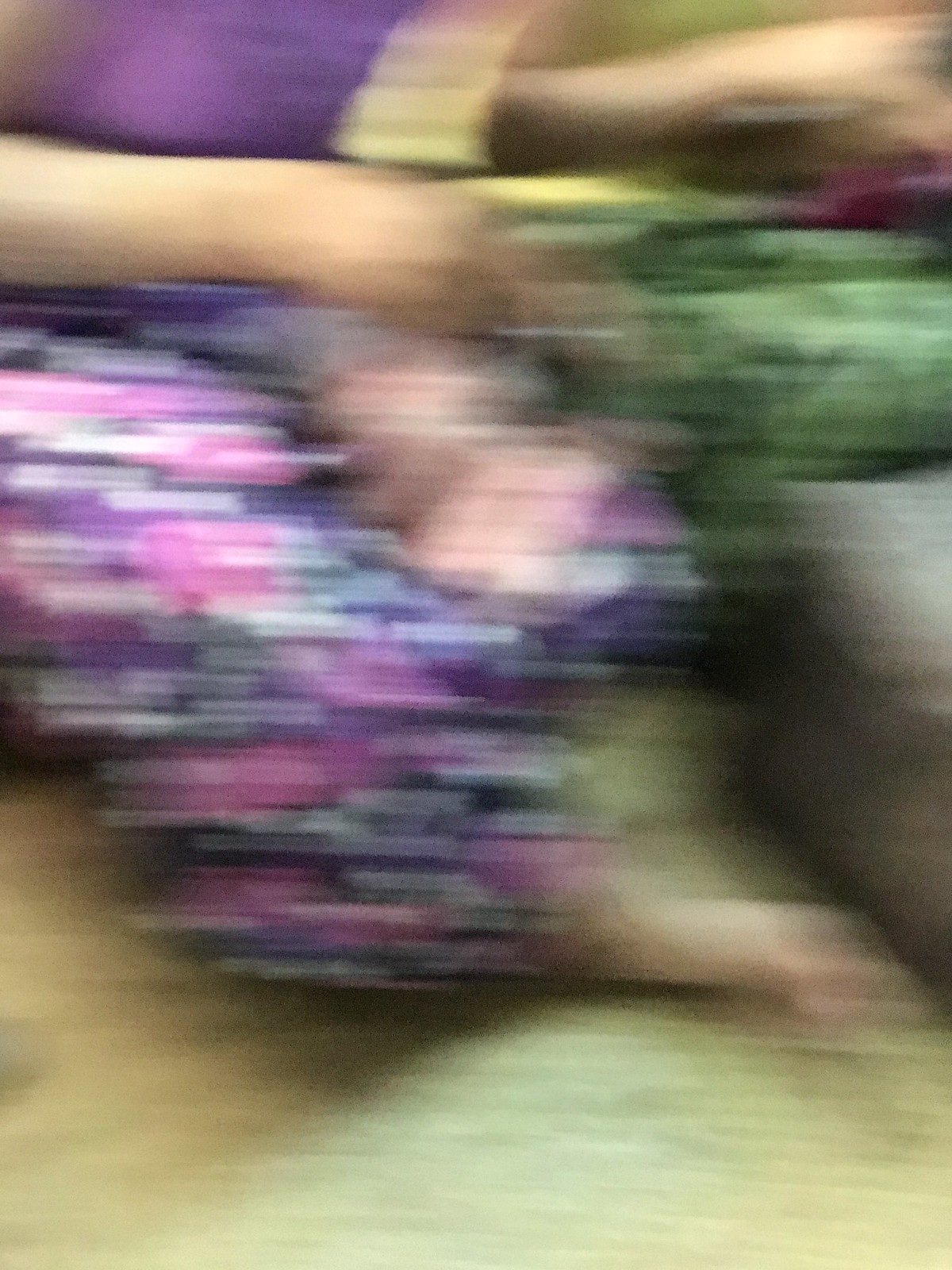The image is an extremely blurry color photograph of a woman sitting on the edge of a couch. She is wearing a bright purple top and multi-colored pants in shades of pink, purple, white, and possibly light blue. Her arms, positioned at the upper left and right-hand sides of the photo, are blurred out. The woman's fair-skinned bare foot is visible at the bottom right of the image, resting on a muted yellow-gray carpet. Next to her foot is a dark gray piece of furniture, which might be an ottoman. She appears to be holding or grabbing a green object. The background includes a brown couch cushion in the right-hand side of the photo.